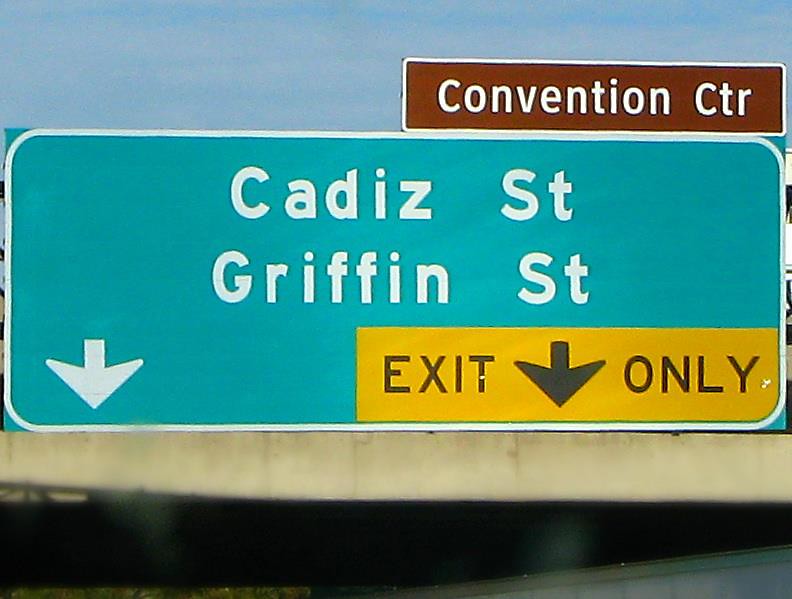The image showcases a prominent freeway sign positioned centrally against a backdrop of clear blue sky. The main sign, a teal-colored panel, displays "Cadiz Street" followed by "Griffin Street" in bold white letters. To the left, a white downward-pointing arrow directs traffic. Adjacent to the right side of the teal sign is a rectangular yellow sign with black lettering that reads "Exit, Arrow Down Only." Above the teal sign, on the right-hand side, there's a smaller rectangular sign with a brown background and white lettering indicating "Convention Ctr" (abbreviated for Convention Center). Beneath the signs, part of the supporting overpass structure is visible, separating the detailed signs from the darker, largely black space below, with a small section of white on the lower right-hand side.